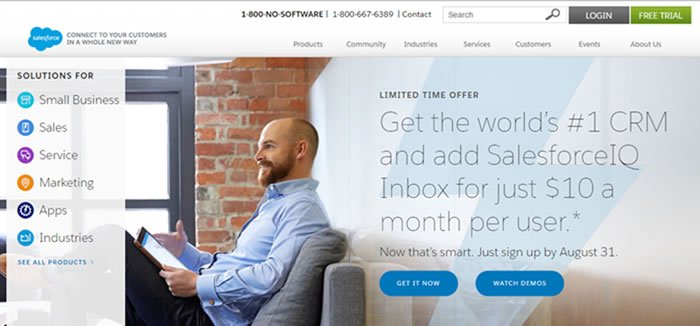The screenshot showcases a comprehensive view of a Salesforce website page. At the top, in bold black letters, the text reads "1-800-NO-SOFTWARE / 1-800-667-6389 / Contact," immediately followed by a search bar and options to log in or start a free trial. Directly below, a navigation bar lists several categories: Products, Community, Industries, Services, Customers, Events, and About Us.

On the left side, the Salesforce logo is prominently displayed, accompanied by the tagline, "Connect to your customers in a whole new way." Beneath this, a vertical menu offers a variety of solutions, including options for Small Business, Sales, Service, Marketing, Apps, Industries, and a link to see all products.

Central to the image is a photograph of a fair-skinned man seated in a gray armchair. He has short, dark hair and a full beard, and he is looking off to the left with a smile on his face. He wears a blue button-down collared shirt and holds a tablet in his hands. The backdrop features a brick wall and a window letting in natural sunlight, contributing to a warm, welcoming atmosphere.

To the right of the photograph, a promotional text reads, "Limited time offer: Get the world's number one CRM and add Salesforce IQ Inbox for just $10 a month per user. Now that's smart. Just sign up by August 31st." Beneath the offer, the call-to-action buttons are displayed in two blue oblong shapes with white lettering: "Get It Now" on the left and "Watch Demos" on the right. The overall image has a wider aspect ratio, making it visually expansive.